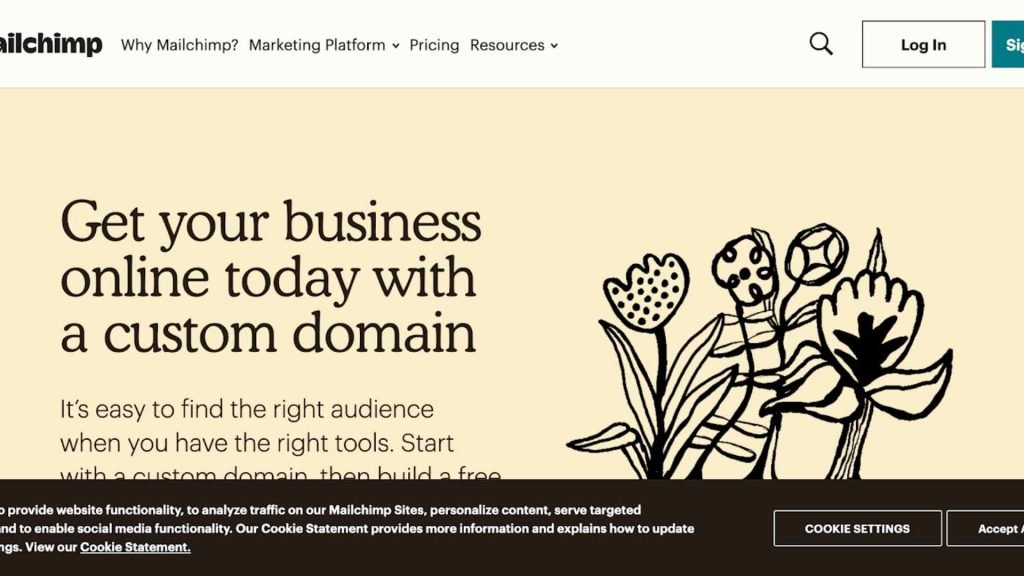A cropped screenshot of a webpage shows a portion of what can be deduced to be MailChimp’s website, though the left edge is cut off, leaving out parts of the brand name. The visible part of the top navigation bar reads: "Why MailChimp", "Marketing Platform", "Pricing", and "Resources." On the top right corner, there is a "Login" button, and a possibly truncated "Sign Up" button. This navigation bar occupies roughly 10% of the image's height.

The remaining 90% of the screen displays a yellowish-peach background. On the left half, large bold text reads, "Get your business online today with a custom domain." Below it, in smaller letters, it says, "It's easy to find the right audience when you have the right tools. Start your custom domain, then build a free..." The right half is dominated by a simple, hand-drawn illustration of flowers. 

At the very bottom of the image, a cookie consent banner is visible, offering options for "Cookie Settings" and "Accept All."